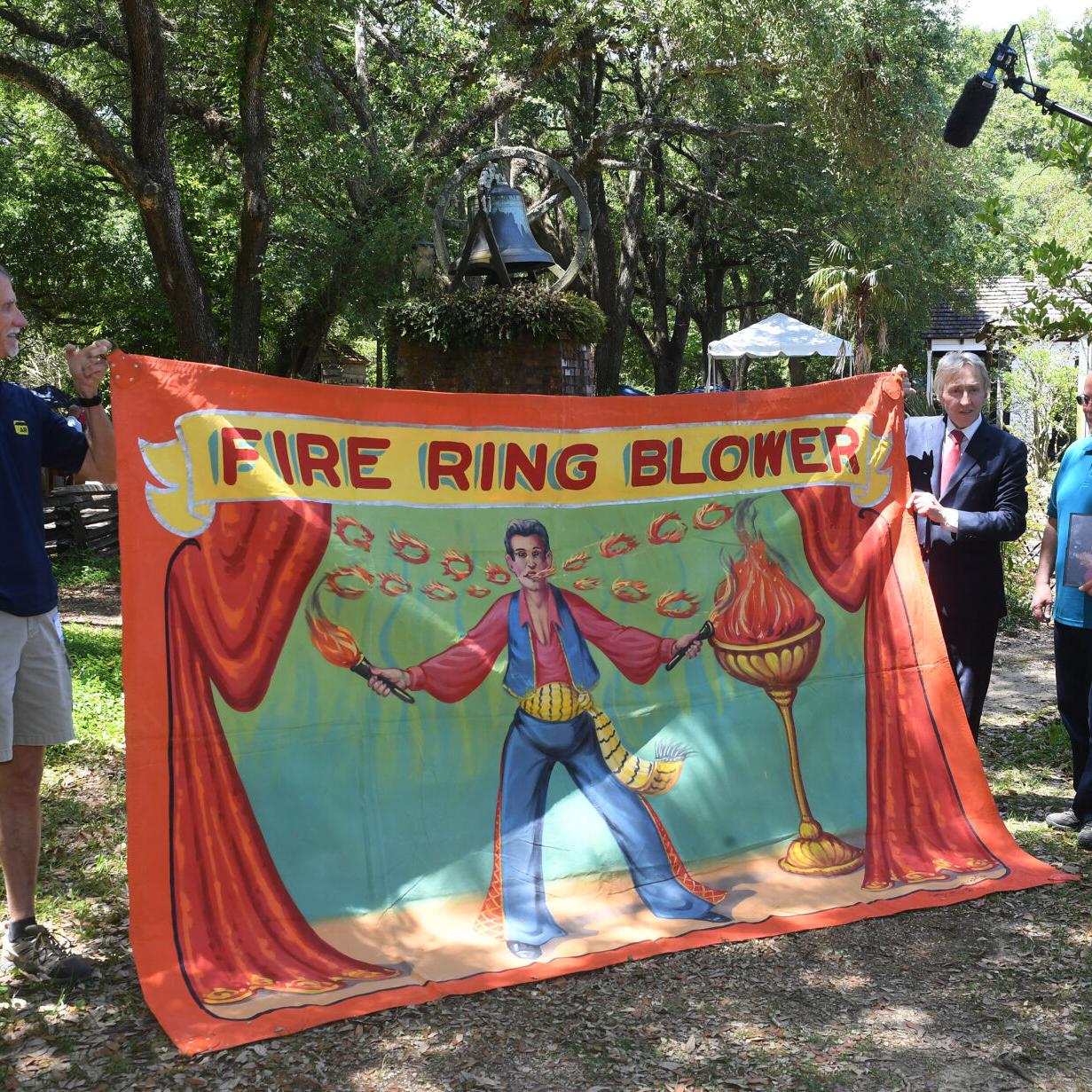In the image, two older gentlemen are holding up a large banner outdoors. The banner prominently features the text "Fire Ring Blower" at the top in a gold color. The illustrated scene on the banner shows a man dressed as a carnival performer, wearing blue pants, a red shirt, a blue vest, and a yellow scarf tied around his waist. He is holding two flaming torches and is depicted blowing rings of fire from his mouth. The background of the banner is a reddish hue, framed by red curtains on either side. Behind the banner, there's a bush with a dark metal bell visible. The setting appears to be a park, evident from the visible trees and an additional gentleman who is part of the setup, possibly due to a visible overhead camera suggesting a recording or news event related to a carnival act.